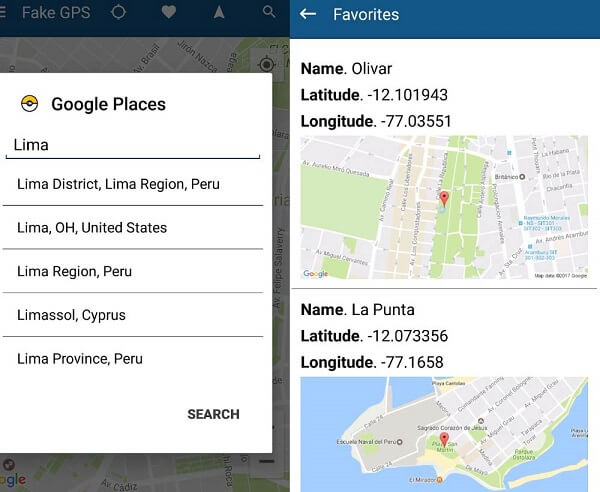Screenshot of a GPS Interface with Fake GPS Overlay

This screenshot depicts a GPS interface ostensibly from Google, although a subdued "fake GPS" watermark in the top left-hand corner suggests that the source may not be authentic. The individual using the service has searched for "Lima," resulting in several location options: Lima District, Lima OH United States, Lima Region Peru, Limassol, Cyprus, and Lima Province Peru.

On the right-hand side of the screen, a list of favorite locations is visible. The first favorite, named "Oliver," has coordinates of latitude -12.101943 and longitude -77.035. Below it, another favorite location named "La Pinta" is listed with coordinates of latitude -12.07 and longitude -77.1658. 

The interface also features a search bar, a white heart icon in the top right corner, and an additional search bar that appears to be for localization purposes, providing versatile options for navigation and location storage.